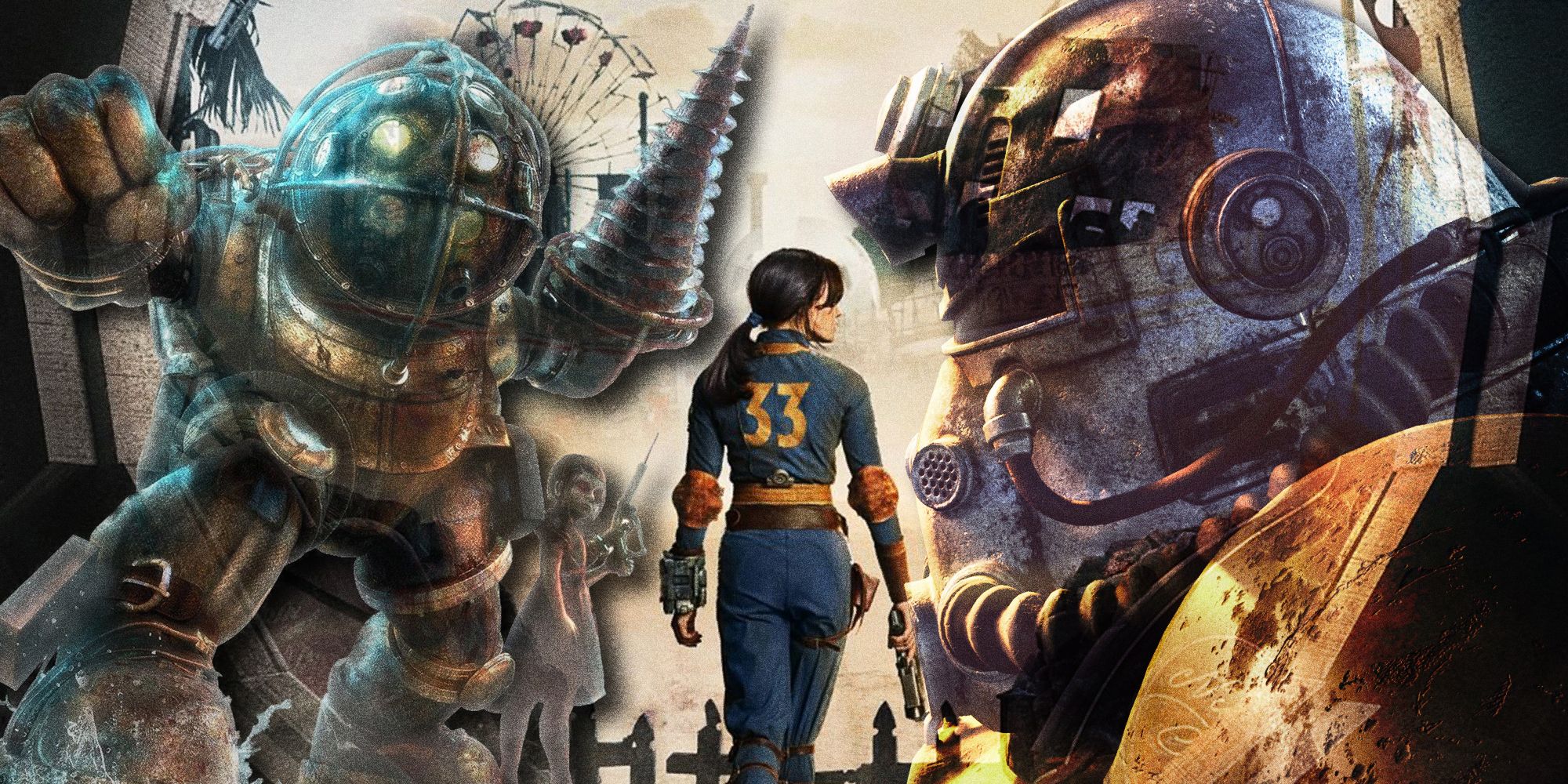This wide horizontal image appears to be a graphic design, possibly from a movie poster. At the center is a female figure with a long ponytail and bangs, her head turned to the right in profile. She is a Caucasian female adorned in a blue long-sleeved uniform and matching pants. Her attire is complemented by brown elbow pads and a gun belt with a holster on her right hip. In her right hand, held down at her side, she grips a firearm. Notably, the back of her uniform features the number "33" in gold lettering.

Flanking the central figure are two menacing figures, possibly enemy combatants or targets she is hunting. The figure on the right resembles a gladiator, wearing a metal helmet with a breathing hose attached and a narrow visor. This figure also boasts metallic shoulder armor, enhancing their formidable appearance. The figure on the left is equally intimidating, equipped with a corkscrew left hand and an oversized metallic right hand, which remains clenched. This character wears a round, clear helmet featuring four white circles, which may serve as eyes, and is encased in an armored suit.

The poster's design reflects a high stakes and action-packed narrative, centered around the central female figure and her adversaries.